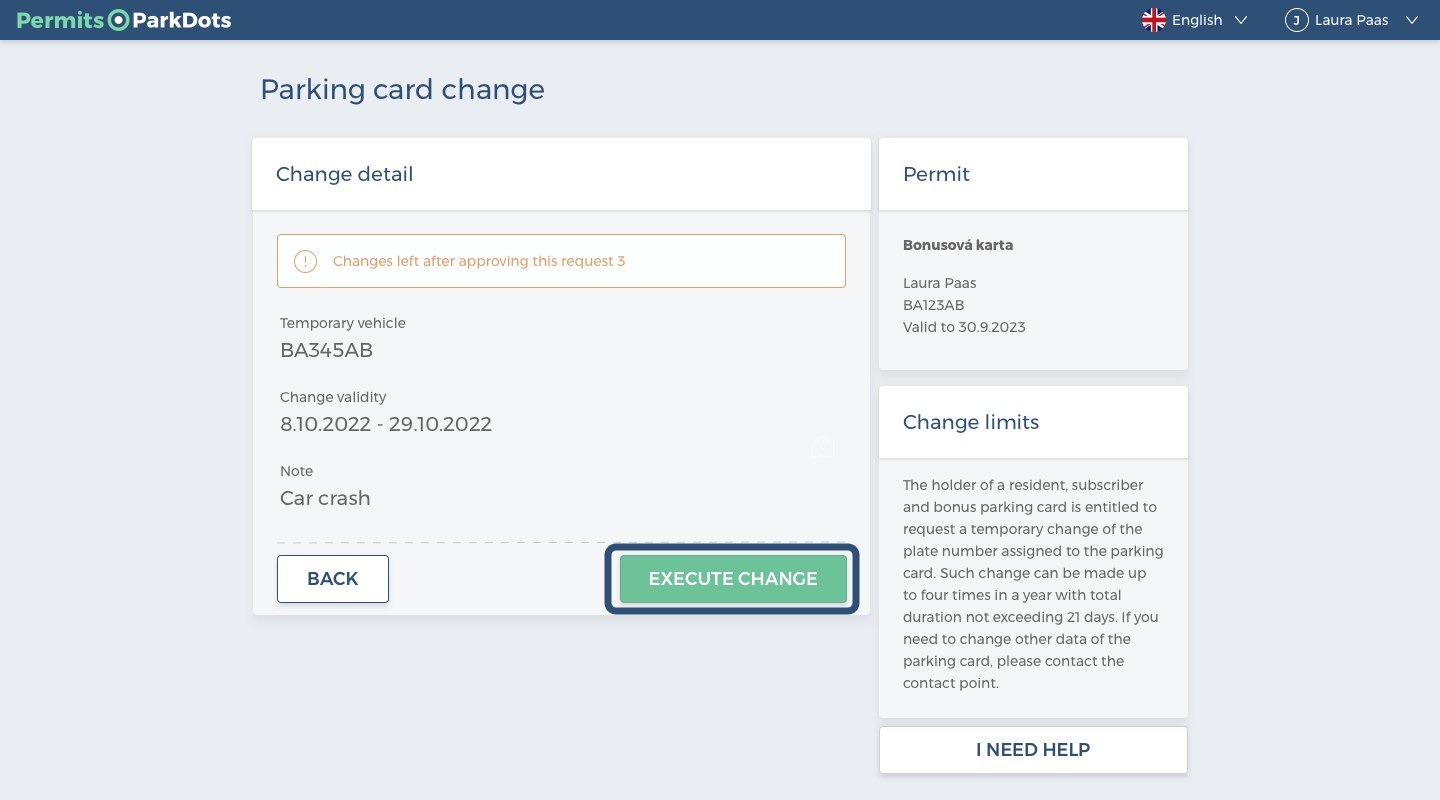This screenshot displays a detailed section of a website related to parking permit management. At the top of the page, a blue bar spans the top 5% of the screen, with the text "permits.parkdots" prominently displayed. The interface is in English, and the user, identified as Laura Paas, is shown in the upper right-hand corner.

The main body of the page is predominantly grey, with various informative boxes and sections. The heading "Parking Card Change" is noted, followed by a subheading "Change Detail." On the left-hand side, there is a detailed section explaining the conditions and options available for changes:

- Charges left after approving this request: 3
- Temporary vehicle: BA345AB
- Change validity: 8.10.2022 - 29.10.2022
- Note: Car crash

On the right-hand side, another detailed section provides the following information:

- Permit: Bonus Cova Carta
- Holder: Laura Paas
- Vehicle: BA123AB
- Valid until: 30.9.2023

Below this, a section titled "Change Limits" explains the policy for changing the plate number assigned to the parking card. Subscribers holding a resident and bonus parking card are entitled to request a temporary change up to four times per year, with each change not exceeding 21 days in duration. 

Additionally, if users need to change other data on their parking card, they are advised to contact the relevant contact point for assistance. At the bottom of the page, there is a conspicuous button labelled "I need help" for users requiring further support.